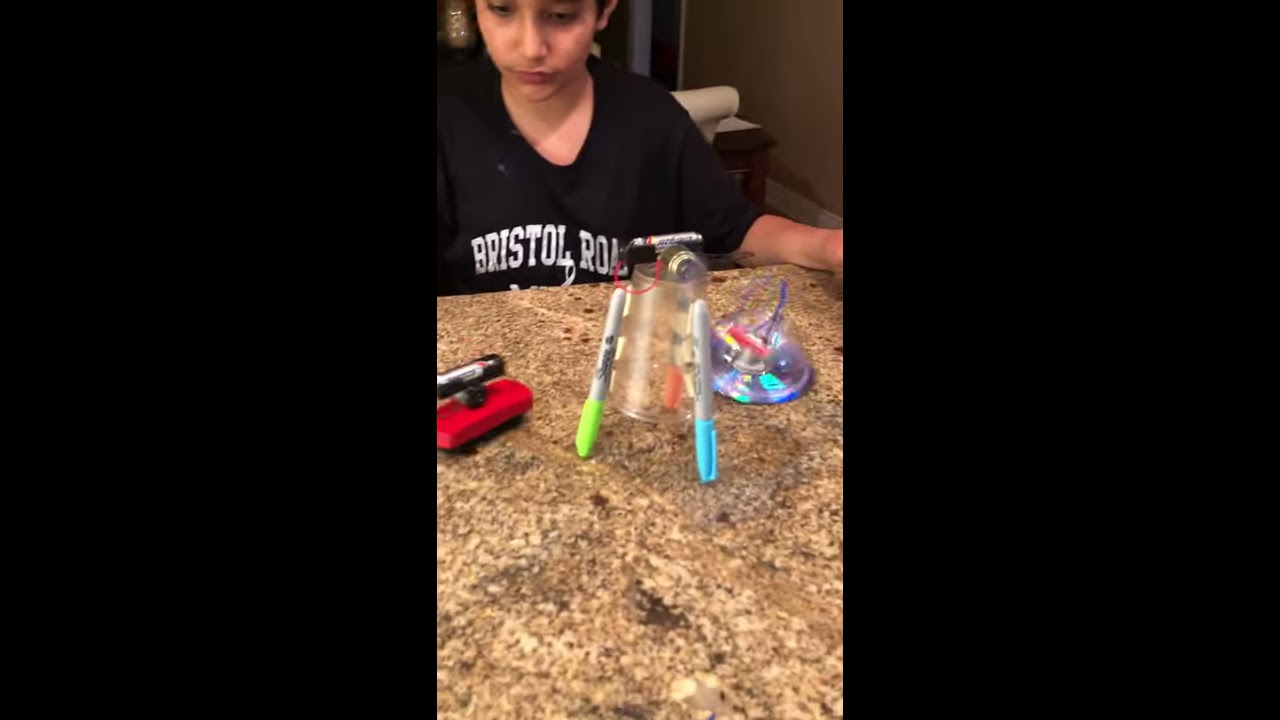An indoor photo shows a young girl, possibly mistaken for a boy, sitting at a kitchen table with a brown and white speckled marble surface, leaning her right arm against it and looking down at an intriguing science experiment she seems to have constructed. She is wearing a black t-shirt with the words “Bristol Road” emblazoned in white letters across her chest. On the table, there is a makeshift robot or contraption that appears to be a combination of various items. This includes a red, remote-shaped object with a small black container holding what looks to be an Energizer battery on top. Next to it, positioned at the center, is an upside-down clear plastic cup supported by three colored Sharpie pens acting as tripod legs; one Sharpie has a lime green cap, another has a light blue cap, and the third, somewhat obscured, seems to have a red or orange cap. At the top of the inverted cup, a small battery with a red wire can be seen. To the right of this setup sits a blue and silver circular item, possibly a CD, gleaming faintly. The background reveals a white towel and a gray wall, situating the setting possibly within a home kitchen environment.